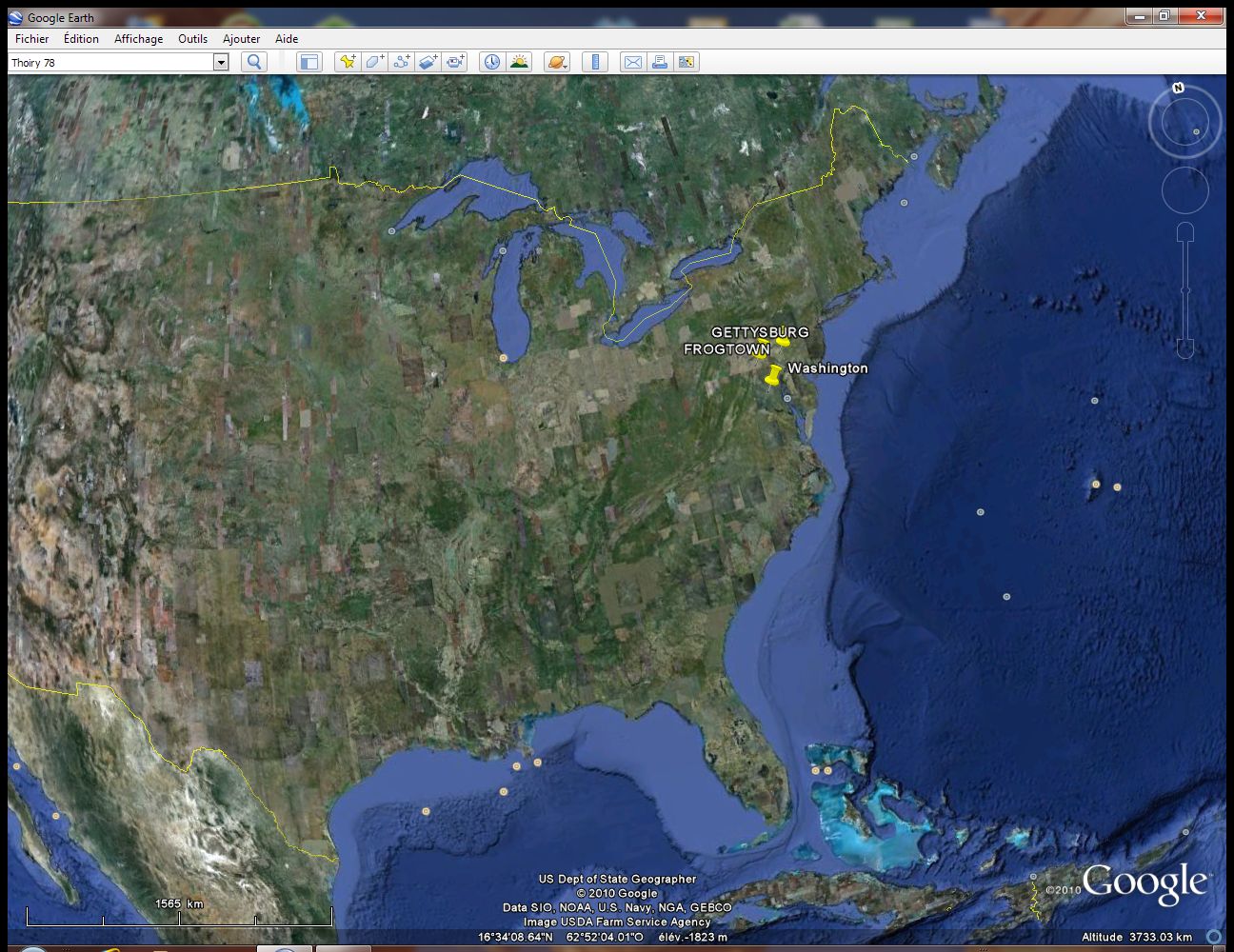The image is a detailed capture of a computer screen displaying a Google Earth map of the United States, extending to parts of Canada and Mexico, with visible oceanic features. The top left of the window prominently displays the "Google Earth" label. Below this, there is a menu bar with various icons, although the text is too small to read clearly. These icons likely allow for the selection of different map layers. Additionally, the menu includes an entry labeled "Theory 78," suggesting different layer options or filter settings.

The map primarily focuses on the East Coast, Southern United States, and Midwest regions. It vividly showcases terrain features such as hills, mountains, lakes, and extensive green vegetation, with the Atlantic Ocean visible to the east. Key pins on the map highlight specific locations, including Gettysburg, Frogtown, and Washington, suggesting an emphasis on historical battlefields.

A thin yellow line marks the border between the U.S. and Canada. At the bottom of the map, white text reads "U.S. Department of State Geographer, Copyright 2010, Google," indicating the source and copyright information. The map scale, located on the lower left side, appears to be in kilometers. Overall, the image presents a rich, textured view of the United States and surrounding areas, framed in a Windows desktop environment.